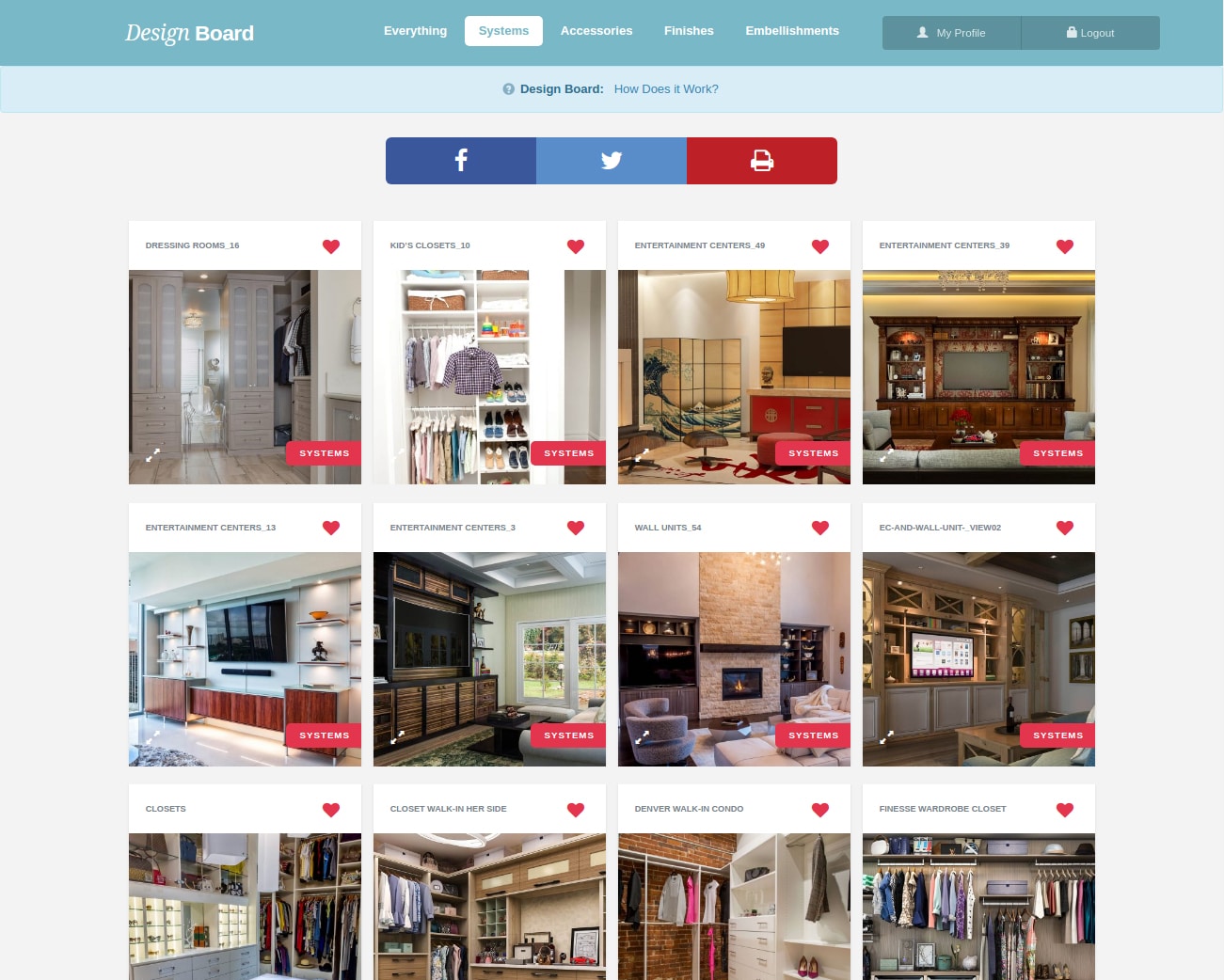Screenshot of a website interface called Design Board. The website title is located at the top left corner. On the right side of the screen, a series of subheadings are present, including "Everything," "Systems," "Accessories," "Finishes," and "Embellishments." To the far right, two buttons labeled "Profile" and "Logout" are visible. Beneath the subheadings, a section titled "Design Board: How Does It Work?" is displayed.

Below this section are three clickable buttons: Facebook, Twitter, and a PDF/save button. The main content area features a 4x3 grid showcasing various types of furniture and finishes. 

- **Top Left:** An image of a dressing room.
- **First Row, Middle:** An image of a kids' closet with children's clothing and shoes.
- **First Row, Right:** An entertainment center featuring a TV in a lit room, adjacent to another entertainment center image showing a room with a couch and TV. 

- **Middle Left:** An entertainment center labeled "Entertainment centers_13" depicting a TV on a wall with various artifacts.
- **Middle Row, Middle:** An entertainment center titled "Entertainment centers_3" showing a TV on a wooden stand next to a window.
- **Middle Right:** Wall units labeled "Wall units_54," showcasing a fireplace situated between several couches.

- **Bottom Left:** A closet displaying an array of clothes.
- **Bottom Row, Middle:** A walk-in closet referred to as "Closet walk-in, her side," featuring various clothes.
- **Bottom Right:** A Denver walk-in condo showcasing a closet against a brick wall filled with clothes.

The final image, labeled "The finesse wardrobe closet," shows a densely packed closet with numerous clothing items.